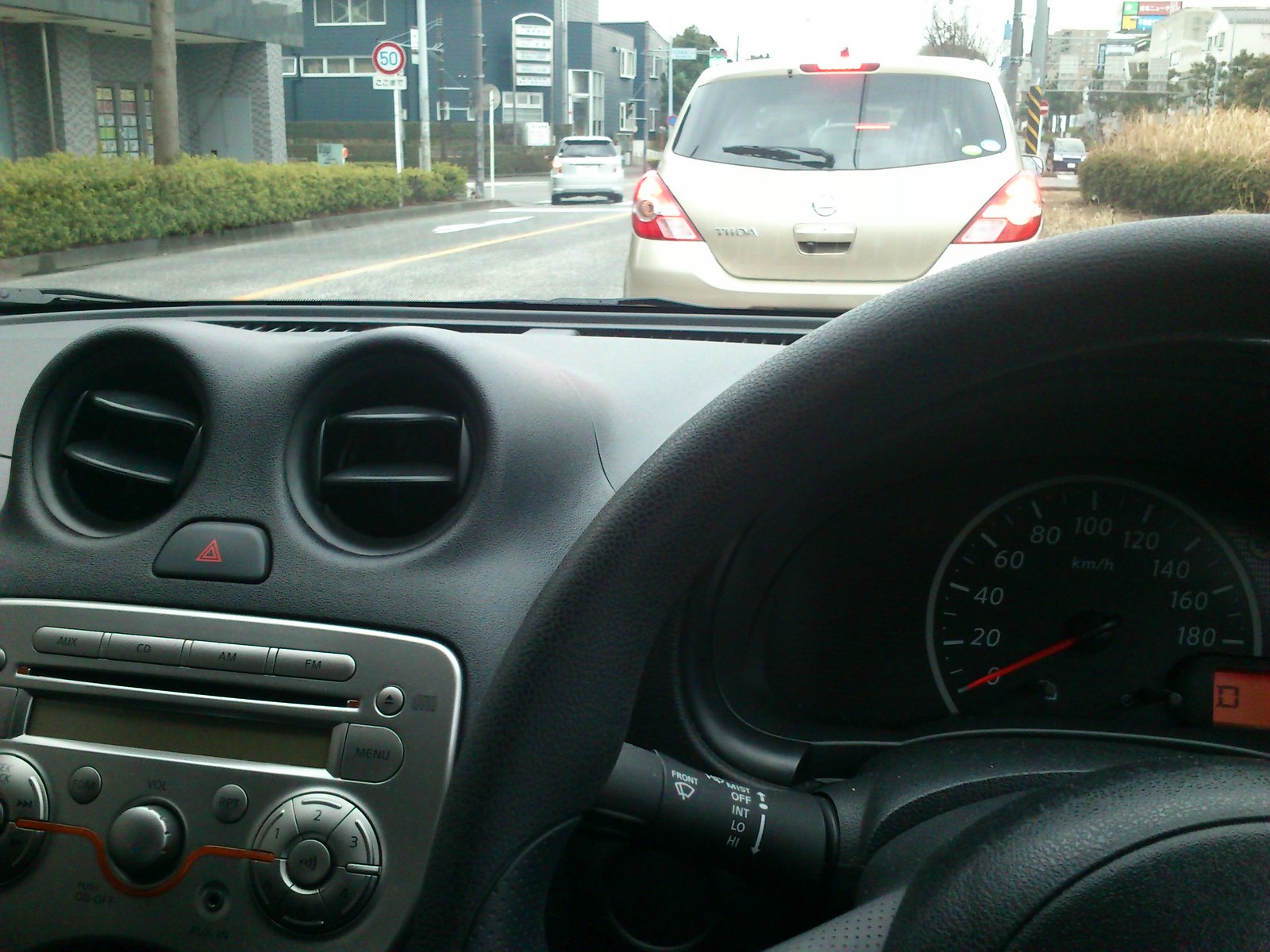The image is a detailed view from inside a right-hand drive car, likely parked or stopped at a light, with the speedometer reading zero. The car's black dashboard features silver and red details, including air conditioning vents, an AM/FM CD radio, knobs, and the steering wheel. Outside, it appears to be a gloomy, overcast day with gray skies. Directly ahead is a small silver car without a license plate, which seems to be making a left turn at an intersection. The road features a yellow center line and multiple lanes, with another lane beside us to the left and an additional turn lane beyond that. To the left in the distance, another silver car is also turning left. Buildings, likely residential with some blue structures, line the street along with untrimmed hedges and visible foliage. Additionally, there are various street signs, including one with a circular shape displaying "50," and electrical or telephone poles can be seen.